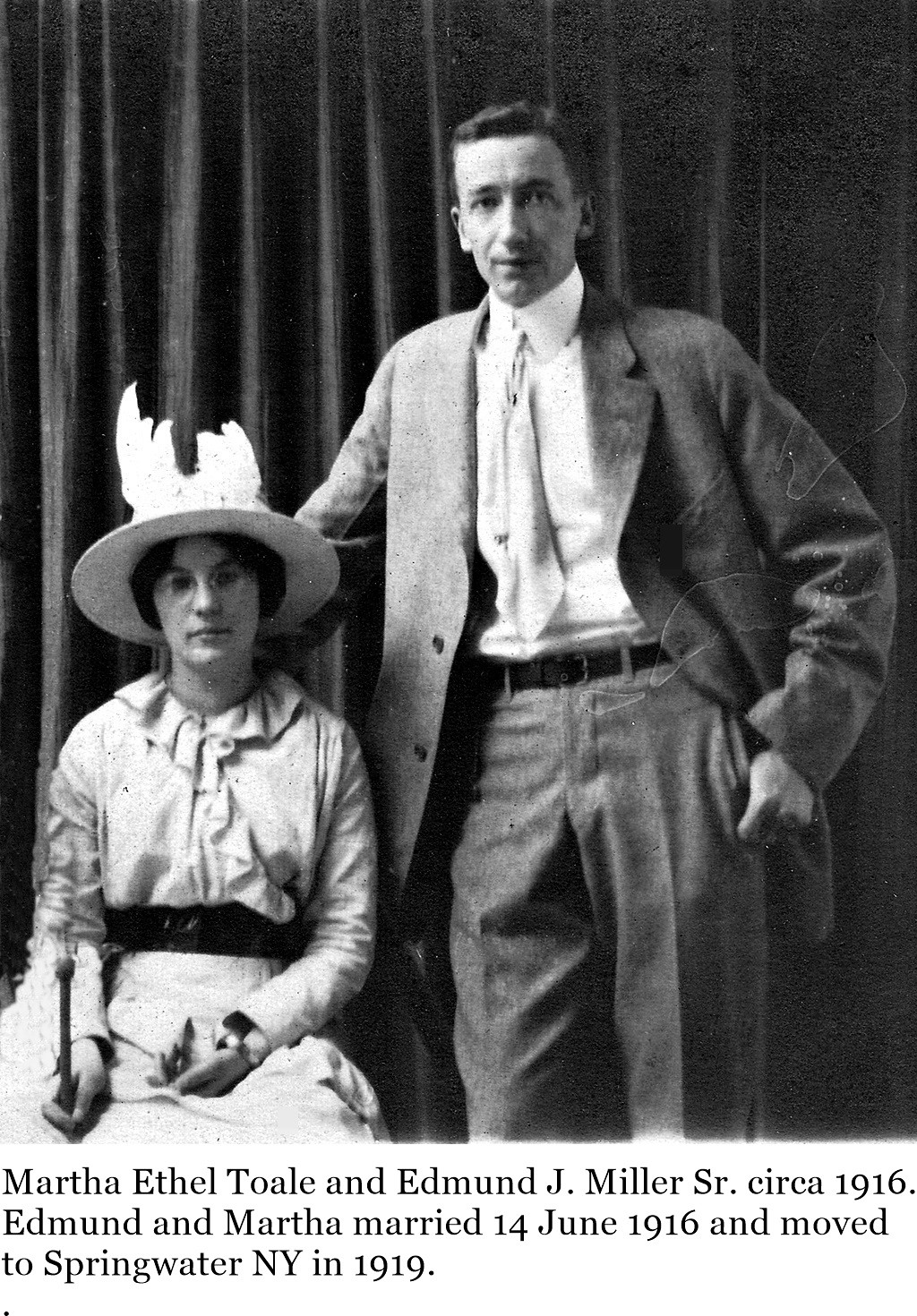This black and white photograph, dated circa 1916, features Martha Ethel Toll and Edmund J. Miller Sr. Martha, seated on the left, dons a white brim hat adorned with feather-like ornaments, along with eyeglasses and a long-sleeve white dress trimmed with ruffles at the collar. She cinches her outfit with a black belt at the waist and holds a metal rod or tool in her hand. Her expression is somewhat bored. To her right, Edmund stands in a gray suit with a white button-down collared shirt and a matching white tie, his right arm partially behind Martha. The photo has a grainy texture, indicating its old age, and a fabric with folds serves as the backdrop. A caption below the image reads, "Martha Ethel Toll and Edmund J. Miller Sr., circa 1916. Edmund and Martha married 14 June 1916 and moved to Springwater, New York in 1919."